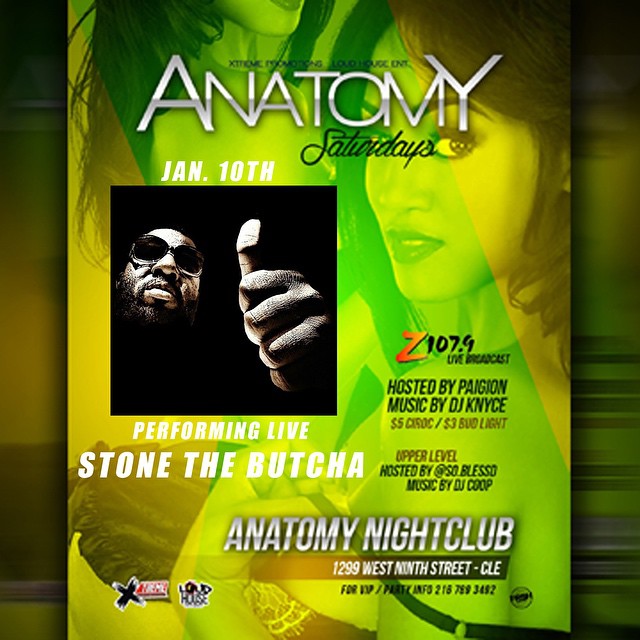The image is a detailed poster advertisement for Anatomy Saturdays, a nightclub event taking place on January 10th. The poster features a gold and green-toned background with two scantily clad women; the one on the right is looking directly at the camera while peeling her bra strap off her shoulder. A central black square photograph shows a man with dark skin, black sunglasses, and a black beard, giving a thumbs up. Bold text above him announces "Performing Live Stone the Butcher." Additional details include "Z107.9 Live Broadcast" and information about special offers like "$5 Ciroc," "$3 Bud Light," and highlights such as "upper level hosted by atso.blessed" with "music by JD Coop." The event is "hosted by Pygion" with music by "DJ Nice." At the bottom, silver text reads "Anatomy Nightclub, 1299 West 9th Street, CLE" (Cleveland), with black text providing contact details for VIP and party information at 216-789-3492.